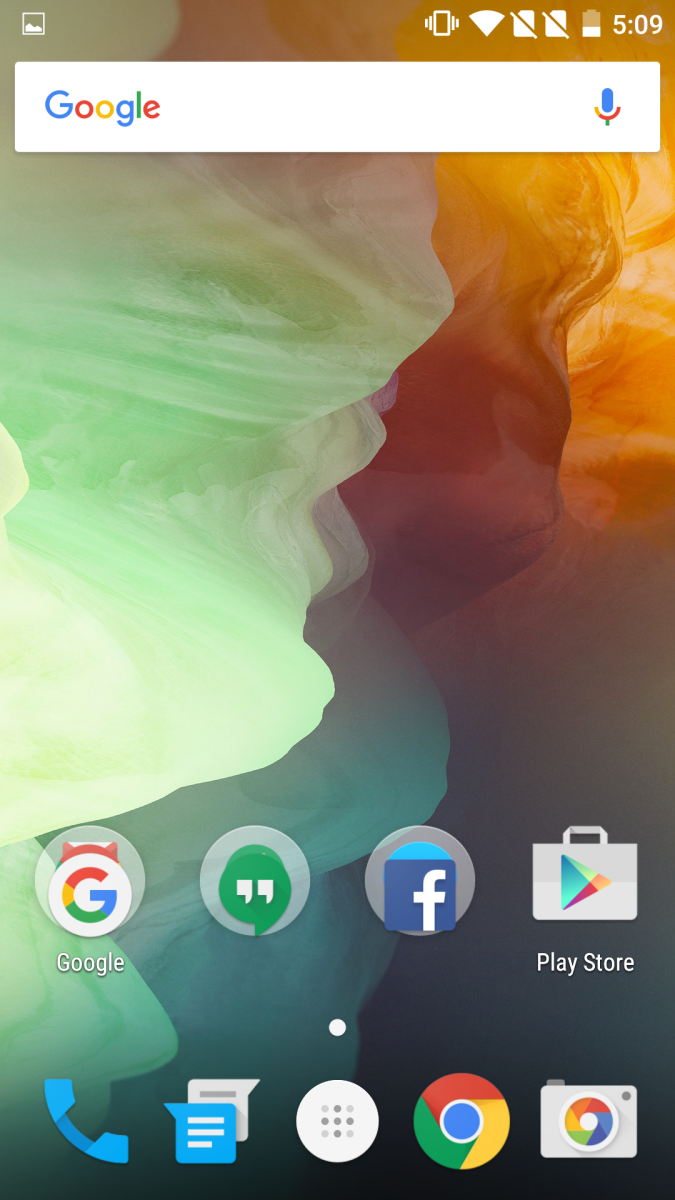This image is a cell phone screenshot showcasing the home screen, complete with various icons and widgets. At the top-left corner, there is the screenshot icon. On the top-right side, one can see the Wi-Fi icon, the battery icon, and the time, which reads 5:09. Dominating the upper portion of the image and slightly cut off at the edges is the Google search bar widget, featuring the Google logo on the left and a microphone icon on the right.

At the bottom of the screen are quick access icons, starting from left to right: the Google Chrome icon, which appears to overlap with another unidentified icon, the WhatsApp icon, the Facebook icon, and the Android Play Store icon. The wallpaper behind these elements is not clearly described but serves as a backdrop to the distinct and commonly used app icons and the Google search widget.